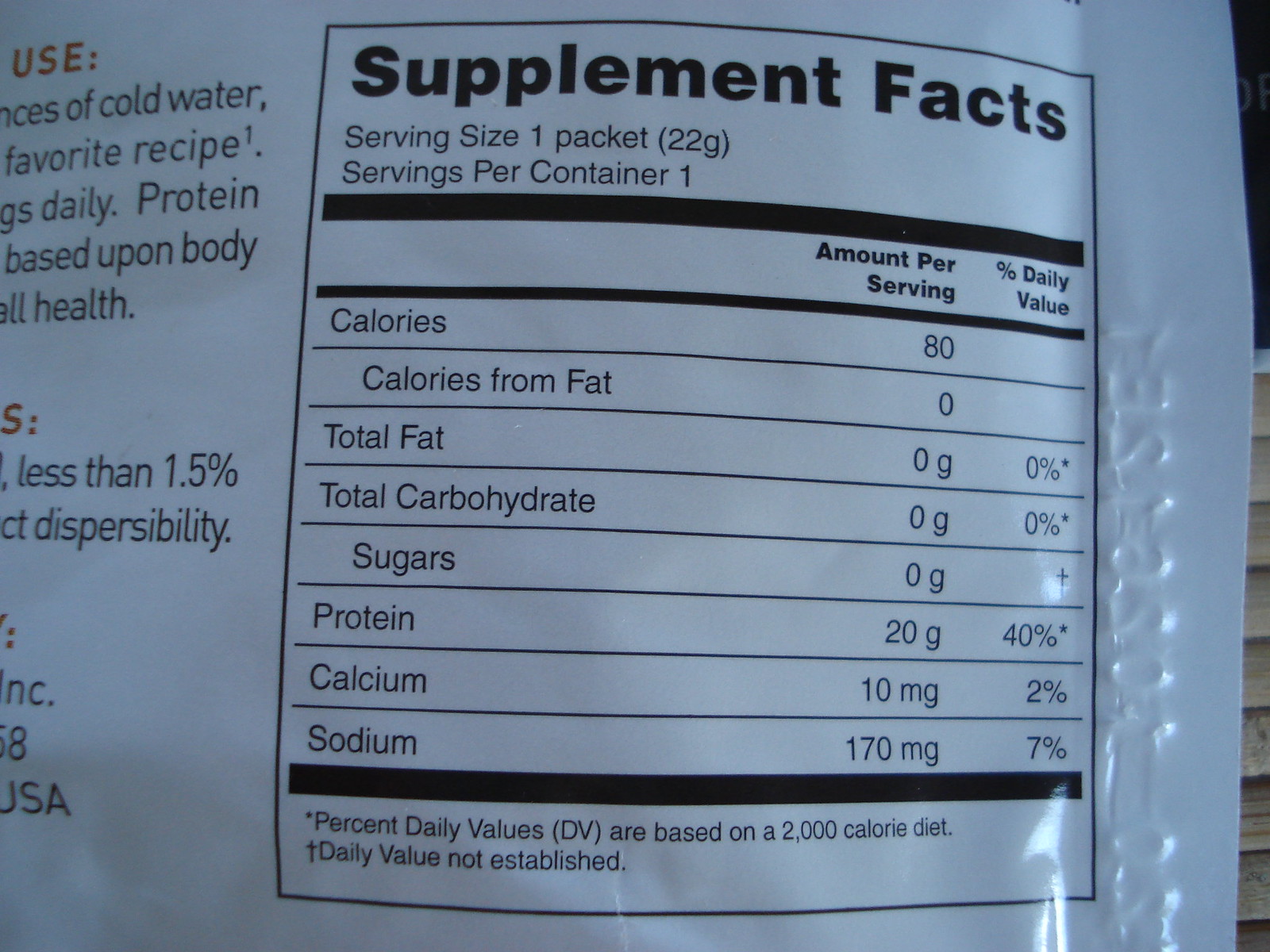This close-up image captures the nutrition label of an unidentified product, likely a protein supplement. The label is clearly marked "Supplement Facts" and provides detailed nutritional information. It states the serving size as "one packet," with "one serving per container." The caloric content is listed as 80 calories, with no calories coming from fat. The label also shows zero amounts for total fat, total carbohydrate, and sugars. Notably, it contains 20 grams of protein, 10 milligrams of calcium, and 170 milligrams of sodium. The partial text visible suggests a mention of protein usage, reinforcing the assumption that the product is protein-based, though other specifics are not discernible from the image.